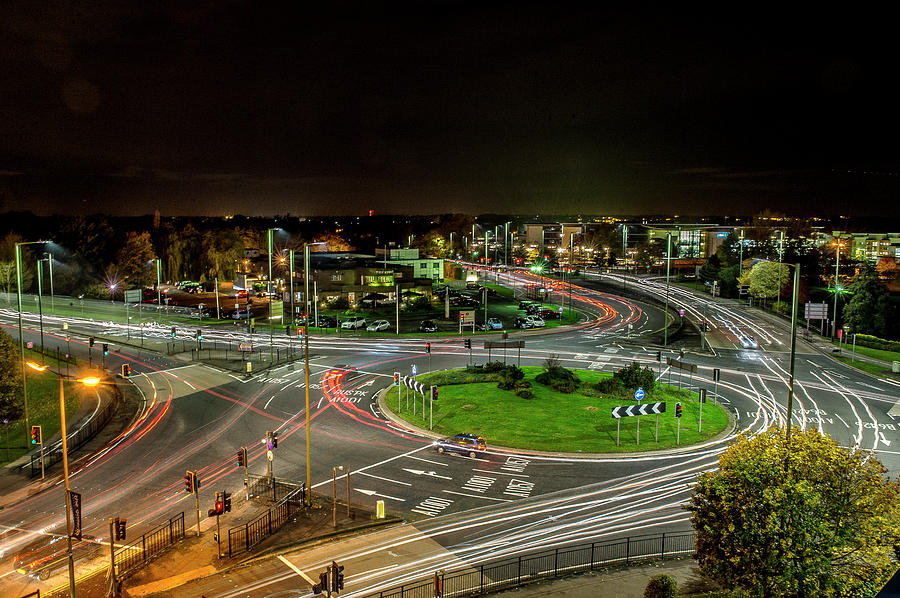This horizontal time-lapse photograph captures a bustling night scene of a large traffic roundabout in a metropolitan area. Shot from a high vantage point, the camera overlooks the roundabout, revealing intricate patterns of light created by the headlights and taillights of numerous vehicles navigating the circle. The most common route, prominently depicted by continuous streams of light, shows cars entering from the bottom and exiting to the left. Surrounding the roundabout are multiple traffic signs with white and black arrows guiding the flow of traffic, and several traffic lights displaying red, yellow, and green signals at each junction. Bordering the roads are walkways with fences, while the center of the roundabout boasts a patch of flat grass with some bushes. The background features a vibrant cityscape with lit buildings and parked cars along the streets, all set against a dark horizon and sky, capturing the dynamic yet orderly essence of city life at night.